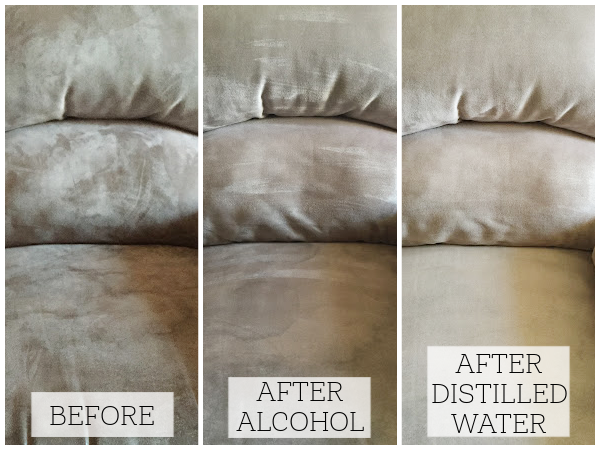The image comprises a three-part sequence showcasing the progressive cleaning process of a beige velvet couch with an initial prominent stain. The first frame, labeled "Before," depicts the couch with noticeable water stains, emphasizing a crackly and unclean texture. The second frame, labeled "After Alcohol," illustrates a slight improvement in softness but still reveals residual stain marks on the cushion. The final frame, labeled "After Distilled Water," presents a dramatic transformation where the couch appears immaculate, as clean as new, devoid of any stains. This visual progression underscores that distilled water is the most effective cleaning method for velvet, delivering superior results compared to alcohol, which leaves the fabric still visibly tarnished.